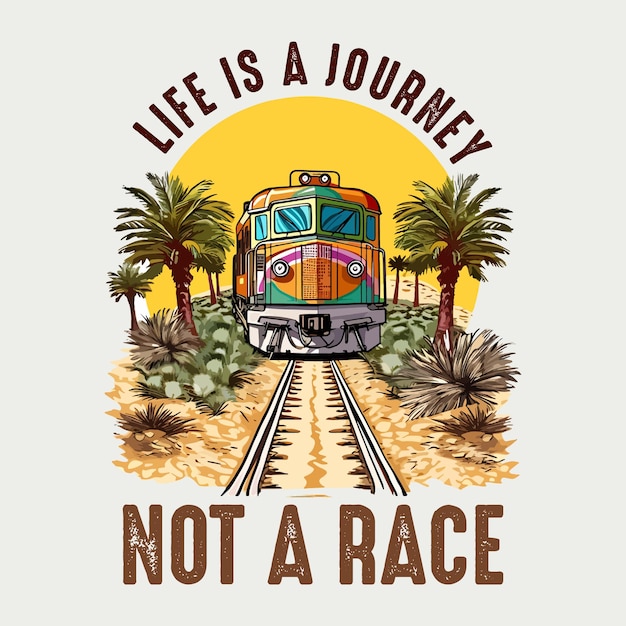This is an inspirational poster set against a light grayish-blue or beige backdrop. At the top, the words "Life is a Journey" are elegantly curved in a dome shape in black and brown letters. Central to the image is a vividly colored passenger train adorned with shades of orange, purple, teal, and red, with silver accents and two bright headlights. The train is moving along tracks that extend towards the viewer, flanked by detailed and lush palm trees and bushes. A radiant yellow semicircle, resembling a sun, provides a vibrant backdrop. Beneath the tracks, the terrain appears sandy and light-colored. At the bottom of the poster, the phrase "Not a Race" is prominently displayed in larger brown and black lettering, reinforcing the inspirational message. The composition, color scheme, and detailed elements create a cheerful and tastefully done image that exudes fun and positivity.